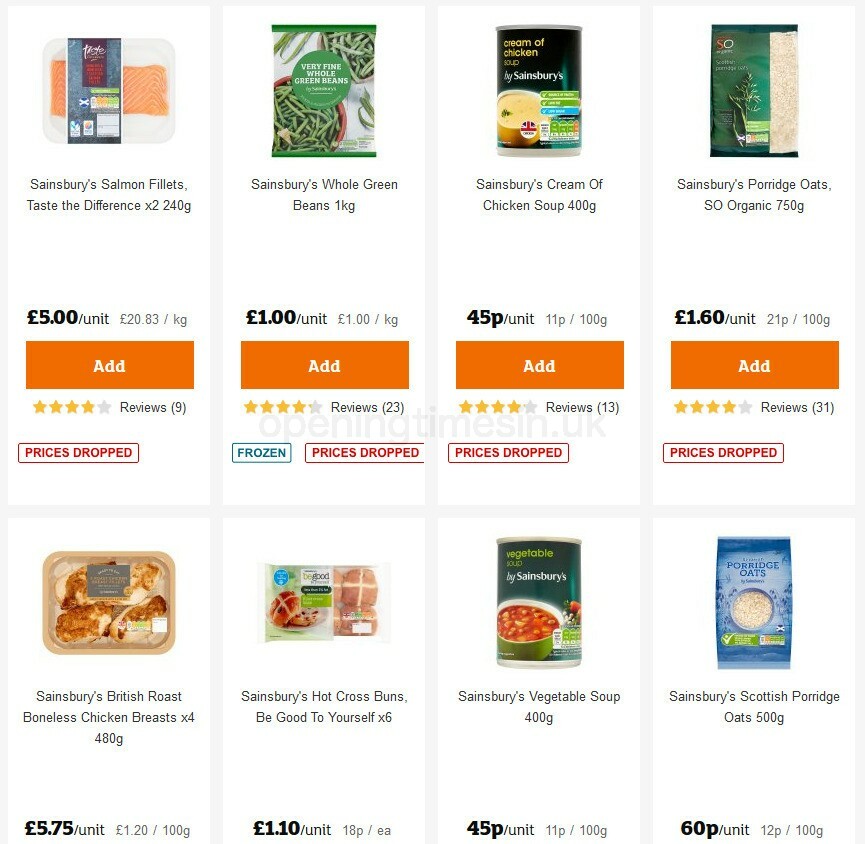This is a screenshot from an unidentified online store, showcasing a product listing against a white background. The products are displayed in two rows, with four items in each row, and the prices are listed in pounds sterling, indicating a UK-based store. Below each product, there's a prominent red "Add" button for adding items to the cart.

Starting from the upper left:
1. **Sainsbury's "Taste the Difference" Salmon Fillets** (2 pieces, 240 grams) priced at £5 per unit or £20.83 per kilogram.
2. **Sainsbury's Whole Green Beans** (1 kilogram) priced at £1 per unit or £1 per kilogram.
3. **Sainsbury's Cream of Chicken Soup** (400 grams) priced at £0.45 per unit or £0.11 per 100 grams.
4. **Sainsbury's Organic Porridge Oats** (750 grams) priced at £1.60 per unit or £0.21 per 100 grams. 

Each product is neatly organized, allowing for easy viewing and selection.